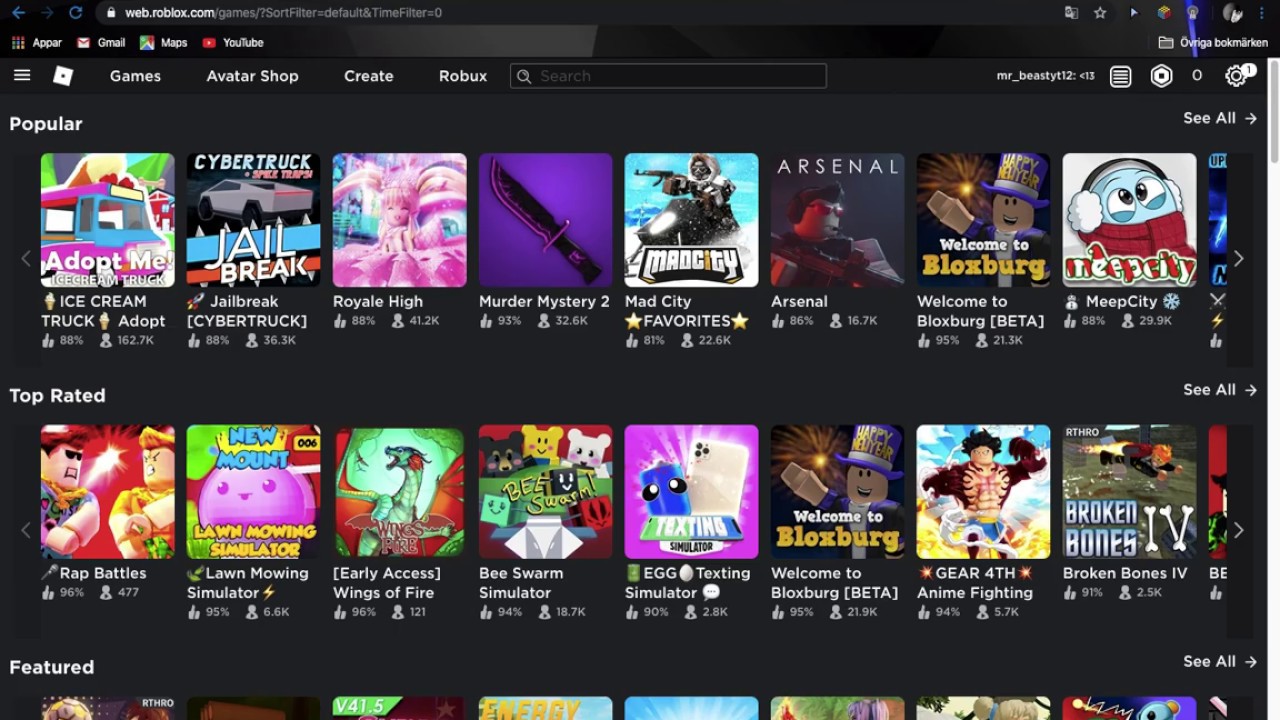The image features a black background with a compact header at the top displaying the website address "webnoblox.com" in small print. On the right, several small icons are visible. A bright blue highlight traverses downward to the next section, which includes various navigable elements: three horizontal lines, a dice icon, links labeled Games, Avatar Shop, Create, Robux, and a search box. Beneath these elements, a box containing lines and a hexagon appears alongside a settings icon marked with a circled number one.

Below this, a "Popular" category showcases several games: *Adopt Me*, *Ice Cream Truck*, *Jailbreak*, *Royale High*, *Murder Mystery 2*, *Mad City*, *Favorites*, *Arsenal*, *Welcome to Bloxburg [Beta]*, and *MeepCity*. One game is partially cut off, and a right arrow suggests more options are available.

Next, the "Top Rated" section is introduced with a right-heading label "See All" followed by a right arrow. Featured top-rated games include *Rap Battles*, *Lawn Mowing Simulator*, *Early Access Wings of Fire*, *Bee Swarm Simulator*, *Egg Texting Simulator*, *Welcome to Bloxburg [Beta]*, *Gear 4th*, *Anime Fighting*, *Broken Bones 4th*, and another partially cut-off game, with an additional right arrow prompting further exploration.

The final section is "Featured," although only the top part of this category is visible. Similar to previous sections, it concludes with "See All" and an accompanying right arrow for additional options.